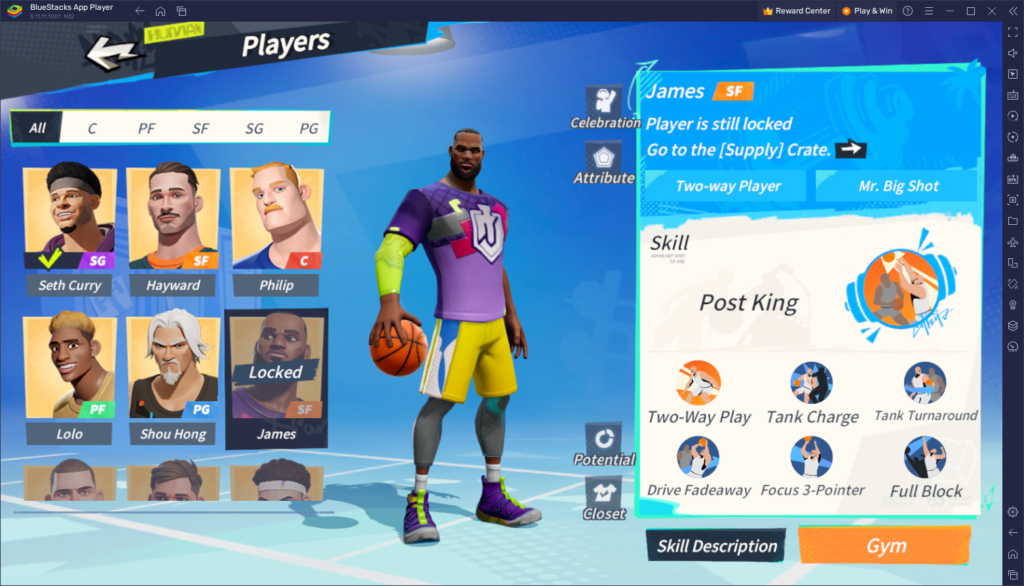The image depicts a graphic interface from a computer or video game, likely associated with a sports theme, given the basketball player depicted. At the top of the screen, there is a black banner displaying the text "Blue's Dax App Player" on the left side. To the right of this text, the banner also features various icons including: "reward center," "play and win," a question mark inside a circle, three vertically stacked lines, a minus sign, a bordered white square with a black center, an "X," and left-pointing arrows.

On the right side of the interface, there are several icons, although their specific details are not fully described. Moving downward, the interface has a black background at the top and transitions into a section on the left side marked by a white arrow. Below this, there is a yellow banner that appears to say "Human," and immediately below it, a black banner with the word "Players" in white text.

The main part of the image features a blue background showcasing a basketball player adorned in a purple shirt, a bright fluorescent yellow elbow sleeve, golden shorts with a design down the side, and purple shoes with white socks. Above the player, there is another banner, black with white text, set against a white background that lists player positions: C, PF, SF, SG, and PG.

The graphic also includes a roster of players with names like Seth Curry, Hayward, Phillip, Lolo, Xiaohong, and James, while the remaining player slots are shown as locked.